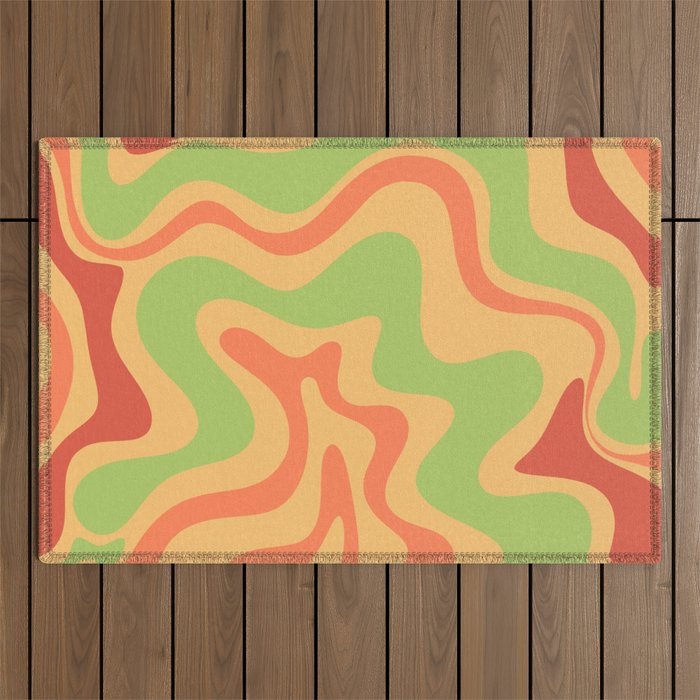The image captures a close-up, overhead view of a vibrant, rectangular piece of art, possibly a placemat or a cloth, situated on an even wooden surface that resembles a floor or a table. The placemat features a groovy, 60s-70s style pattern comprising curvy, wave-like lines that span the entire piece. The colors used include various shades of pink—such as light pink and salmon—dark red, a light green, and beige. These colors are arranged in a sequence featuring darker reds, beige, green, and pinkish hues. The composition's attention to detail reveals a black stitching lining along the edges of the placemat. With the focus solely on the placemat against the wooden backdrop, the photograph is devoid of any other elements or people, emphasizing the intricate design and vibrant colors of this artistic cloth.